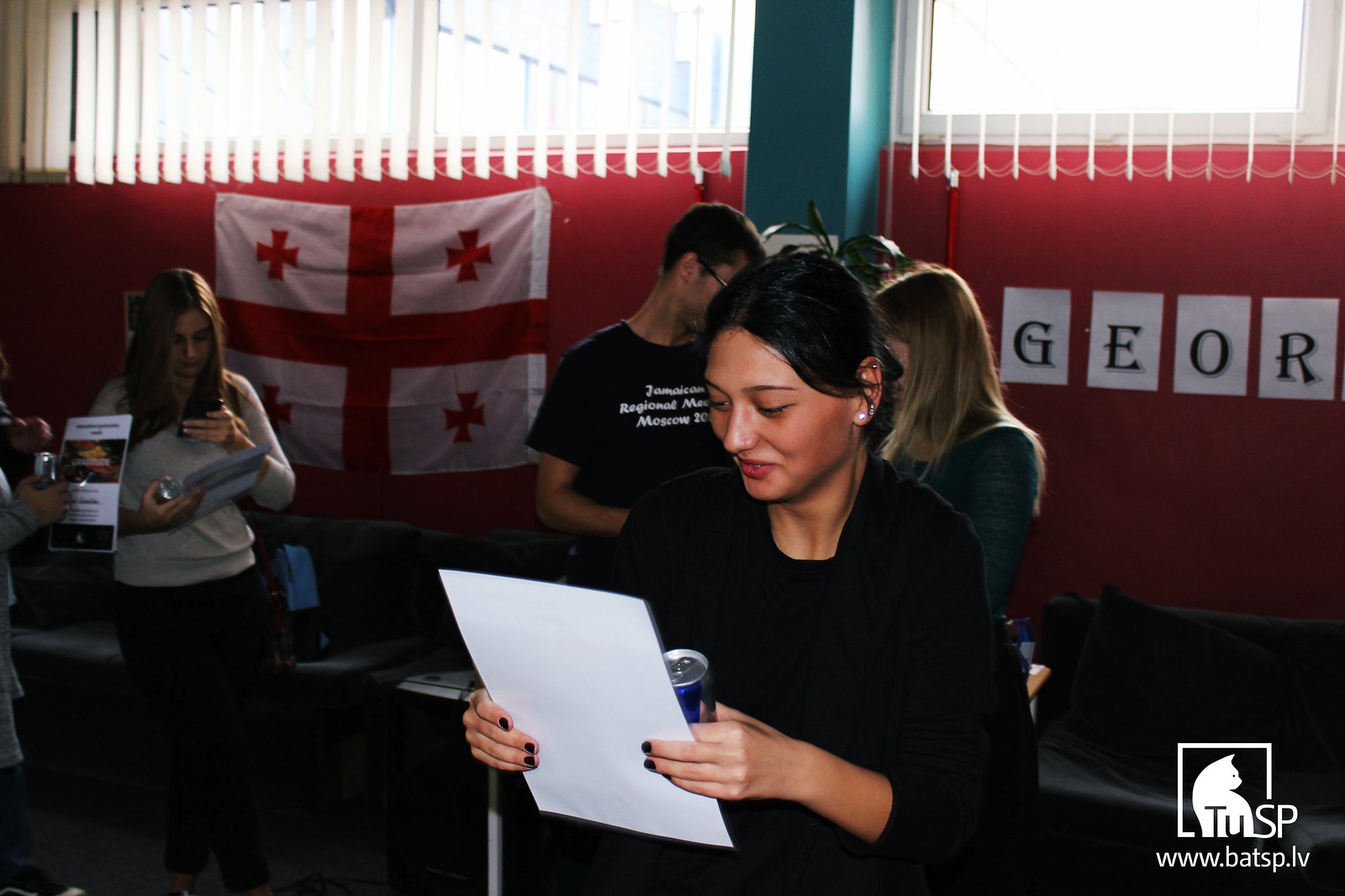In this detailed color photograph taken indoors, the central focus is on a young woman of possible mixed or ethnic descent. She has dark hair pulled back, slightly darker skin, and is wearing a black blouse. Her black-polished fingernails are visible as she holds a white A4-sized piece of paper in her hands, which she is looking at and smiling, suggesting she's happy with its contents. In her other hand, she holds a canned energy drink.

To her right, partially visible, is a young man wearing a black shirt with white writing that includes the word "Jamaican." He is wearing glasses. To her left, a young woman with dirty blonde hair is clad in a green shirt. 

Behind this trio is a red-painted wall featuring several white flags with red cross symbols and pennant letters spelling out G-E-O-R. A pair of windows with open blinds sit above the wall. In the bottom right corner, there's a logo in white with the text "T-U-S-P" and the URL "www.batsp.lv.” The image captures a realistic scene likely set in a banquet or meeting hall, blending elements of Photographic Representationalism Realism.